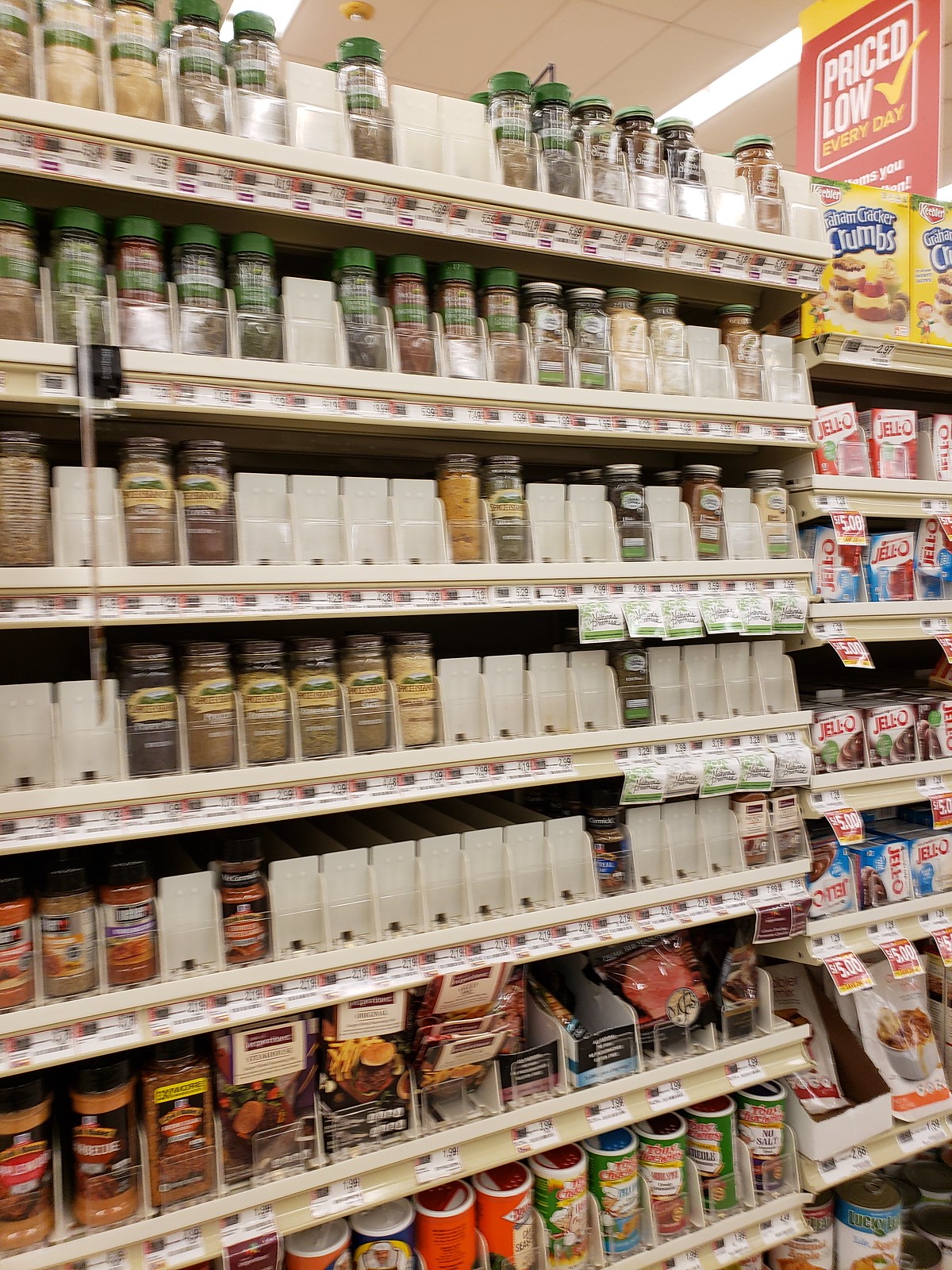The image captures a multi-leveled store shelf dedicated to an assortment of spices and various baking products. The primary section of the shelf contains seven visible levels dedicated to spices, with a barely visible bottom shelf. 

The top two rows predominantly feature clear glass spice jars with green lids, arranged meticulously. Moving down, the next two middle rows showcase spices in more square-shaped containers with brown lids, contrasting the rounded jars above. The fifth shelf, counting from the top, holds a variety of round spice containers with black lids and multicolored labels, although the image's slight blurriness obscures the specific names of these spices.

There are signs of spices running out, as several slots are empty, displaying just the underlying white plastic placeholders. At the base of the spice section, larger canisters of spices or similar products are visible, indicating a broader range of quantities available.

To the right side of the image, a different section of shelving begins. The top shelf houses boxed graham cracker crumbs. Below this, three shelves are stocked with boxes of Jell-O in various flavors, organized neatly. The bottom shelves contain assorted packages, though the image's angle and resolution make it difficult to discern the specifics of these items.